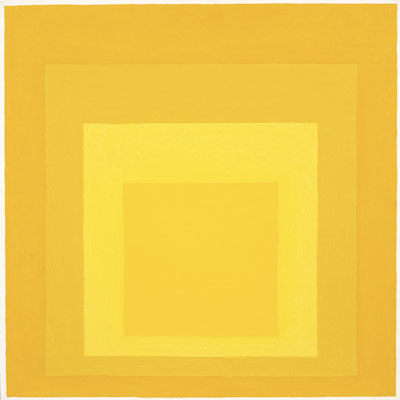This is an abstract, square-shaped oil painting on a white canvas base, featuring a series of concentric squares, each painted in varying shades of yellow and gold. The painting starts with an outermost square in a dark mustard yellow, forming a nearly complete border around the canvas, giving the appearance of a faux frame. Inside this, there's a progression of squares: the next is a lighter mustard yellow, followed by a pale yellow square, then another mustard-colored square. The innermost square, slightly off-center towards the bottom, is painted in a darker gold shade. The shifting tones of yellow and gold create a captivating visual effect, emphasizing the abstract nature of the work. The piece has no text or signature, focusing purely on the interplay of color within the geometric shapes.